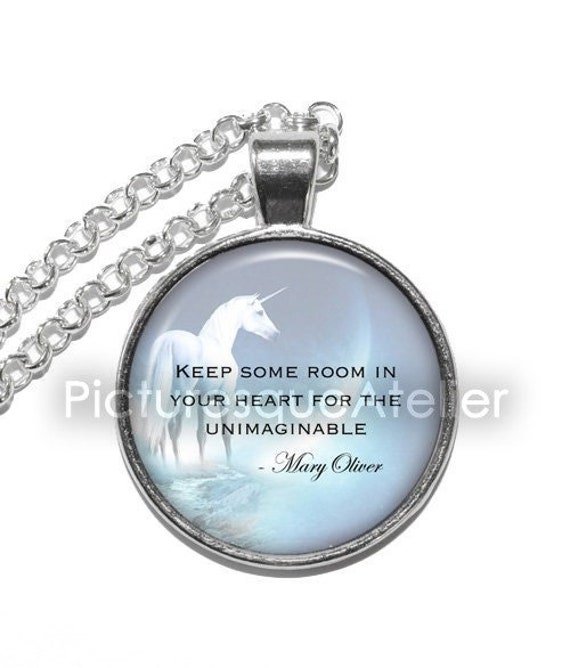This close-up product photo of a pendant necklace, captured against a white background, showcases the intricate details of the jewelry. The pendant features a silver tone ring that frames a captivating image of a white unicorn facing right, standing against a glowing grey or purple backdrop that resembles a beach or water. Prominently displayed across the unicorn image is a motivational quote that reads, "Keep some room in your heart for the unimaginable," attributed to Mary Oliver in cursive font. The pendant hangs from a delicate silver chain composed of small circular links, a portion of which trails off to the left side of the image. The photo is watermarked with "Pitcher-esque Atelier" in white text across the center, subtly indicating the source of the jewelry.